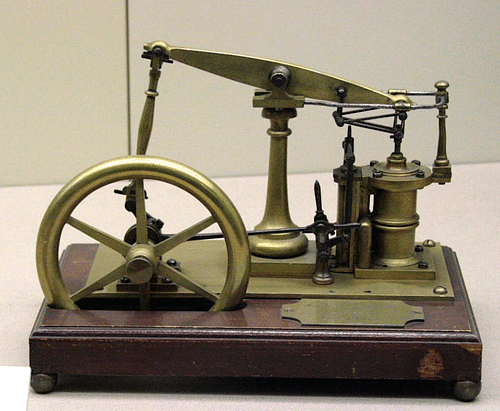This photograph captures what appears to be a meticulously maintained, antique sewing machine, manufactured from a polished, greenish-brass material. The machine is affixed to a small wooden base and features tiny wheels underneath, suggesting mobility. It prominently displays a large wheel on the left side, connected to a hammer-like apparatus which drives the sewing needle. A smaller hydraulic system or scale-like component is situated on the right side, hinting at a more complex mechanism. The entire setup rests on a white table against a white wall, indicating it could be part of a museum exhibit, given its well-preserved condition that suggests it is over 100 years old. This intriguing piece evokes the early mechanisms of industrial sewing, showcasing both functionality and craftsmanship.